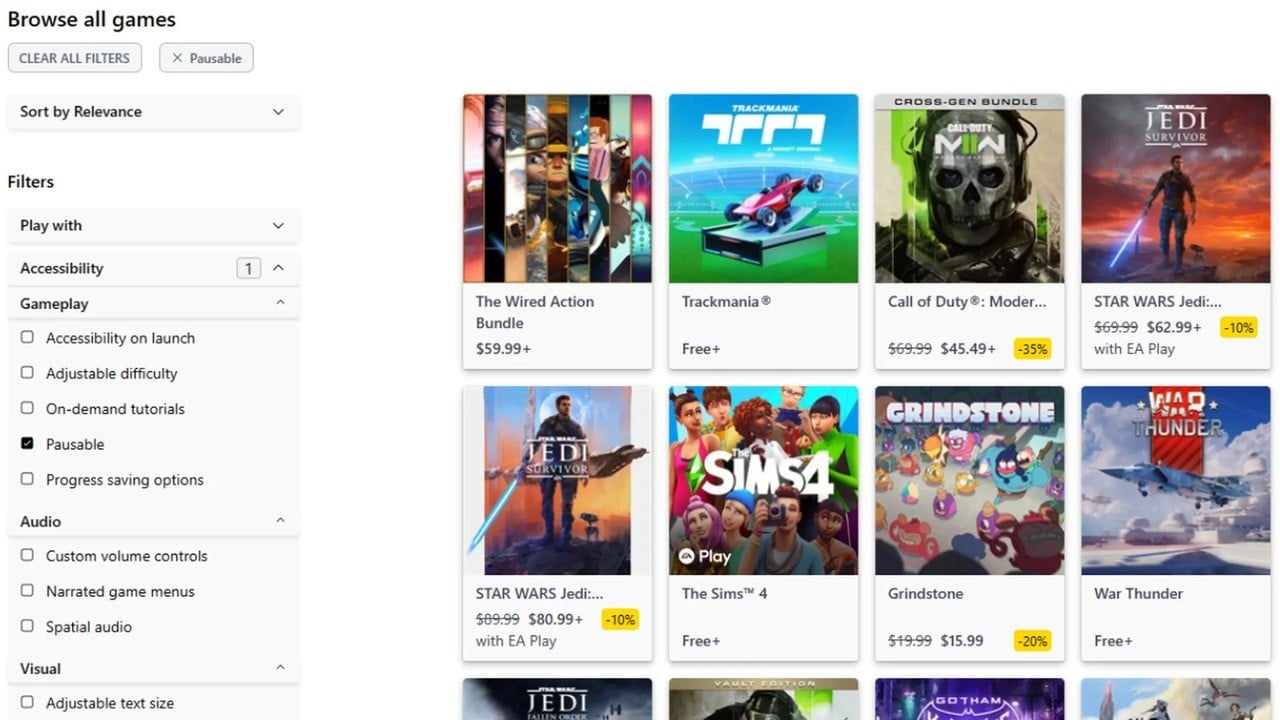The image depicts a detailed video game homepage interface. In the top left corner, there is a black "Browse All Games" banner. Below it, there is a "Clear All Filters" button. Adjacent to this button, there is a "Pausable" label accompanied by an "X" icon. 

Underneath, there's a "Sort by Relevance" drop-down menu followed by a "Filters" section. Within this section, a "Play With" drop-down menu is available, succeeded by an "Accessibility" option, marked with a number "1" icon, and featuring an upward-pointing drop-down arrow.

Further below, there's a "Gameplay" section with an upward-pointing drop-down arrow. This section contains five checkboxes, the first of which is labeled "Pausable" and is checked off. At the bottom of this section, an "Audio" label appears with an upward-pointing drop-down arrow.

Beneath the "Audio" section, the list includes "Custom View Controls," "Narrated Game Menus," "Special Audio," each accompanied by checkboxes. Finally, at the very bottom of the image, there is a "Visual" label featuring an "Adjustable Text Size" option.